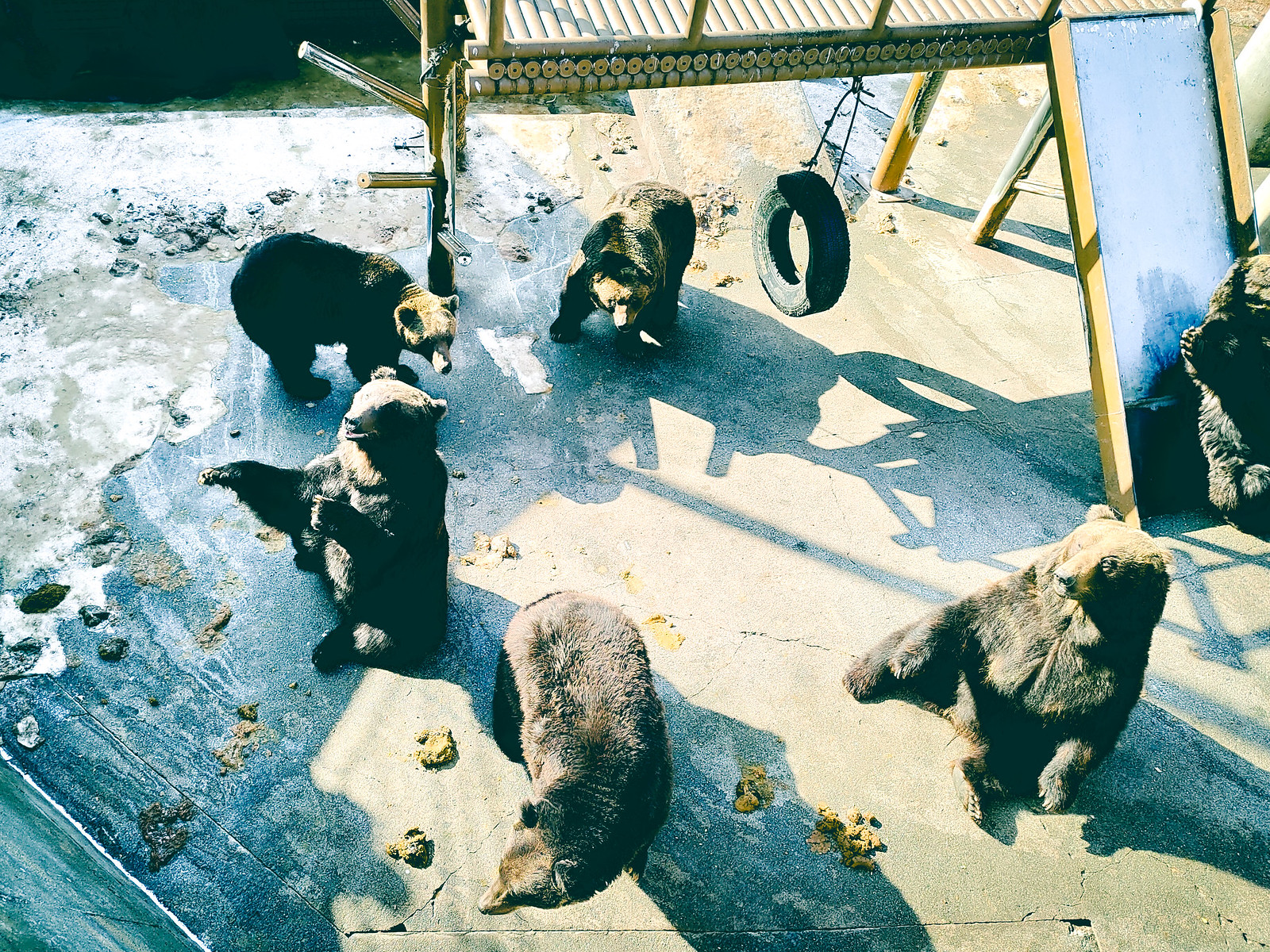This overhead image depicts a group of six bears in what appears to be a playground within an enclosure, likely at a zoo or conservancy center. The playground features a wooden structure with multiple levels, a large slide on the right, and a tire swing. The bears are scattered around a concrete floor that's littered with poop. Towards the top left, there's a mix of snow, ice, and some grass. One bear appears to have just gone down the slide, evident by its shadow and partial view on the right. Another bear is sitting on the concrete, while one is on all fours navigating between the piles of poop. A third bear seems to be looking up at the fence with its hands raised, possibly interacting with a visitor. The remaining bears are either walking around or near the tire swing, engaging with their environment.